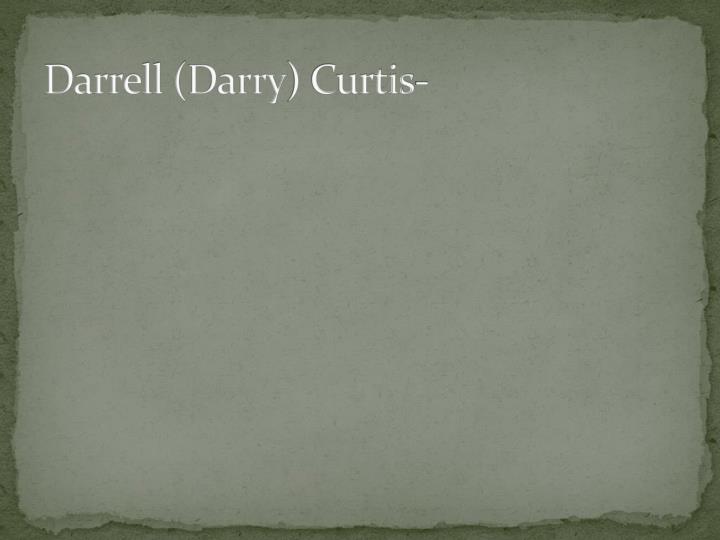The image features a computerized slide with a predominantly green color scheme. The centerpiece is a light green textured area, speckled with dark gray dots, giving it an aged, worn look. This light green section is framed by a darker green border with uneven, jagged edges, evoking the appearance of stone or tattered pages. In the top left corner, there is white text that reads "Daryl (Dary) Curtis-", with the first letter of each word capitalized. The overall design resembles the introductory slide of a PowerPoint presentation, possibly for a school project, and implies an introduction to a character or person.